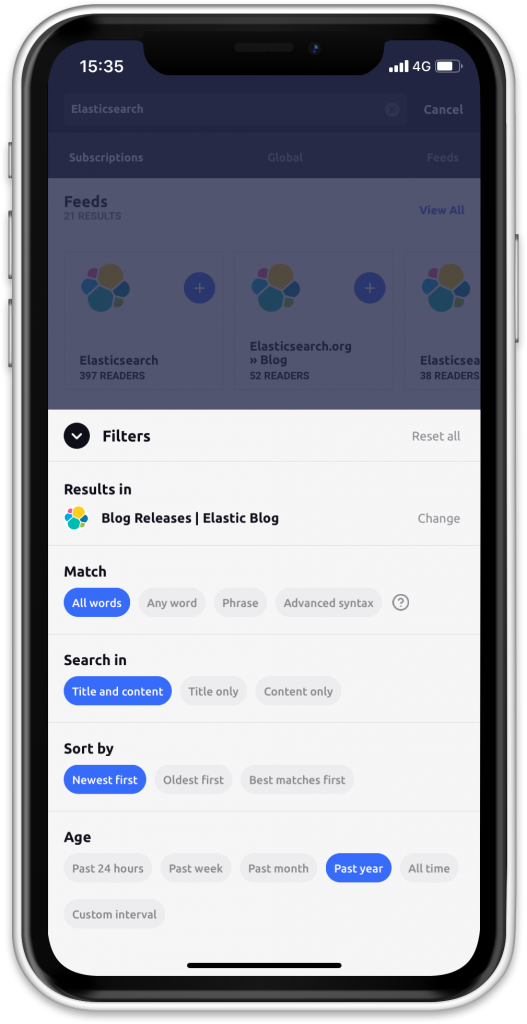In the image, we see a smartphone displaying a user interface. The status bar at the top indicates it is 15:35 or 3:35 PM, with the phone connected to a 4G network, full service bars visible, and a battery icon suggesting ample charge. The left side of the phone features a notification silence switch, while the right side houses the volume up, volume down, and power buttons.

The screen shows a search functionality with "Elastic Search" typed into the search bar at the top, accompanied by a cancel button to its right. Just beneath the search bar, there are three tabs labeled "Subscriptions," "Global," and "Feeds."

In the "Feeds" section, the interface indicates "21 Results" on the left side and a "View All" button on the right. Following this, we see a list of search results: the entry "Elastic Search" with "397 readers," the "ElasticSearch.org blog" with "52 readers," and a partially cut-off entry also showing "Elastic Search" with "38 readers."

At the bottom half of the screen, a pop-up labeled "Filters" is visible, offering options to change "match," "search in," "sort by," and "age" to refine the search results.